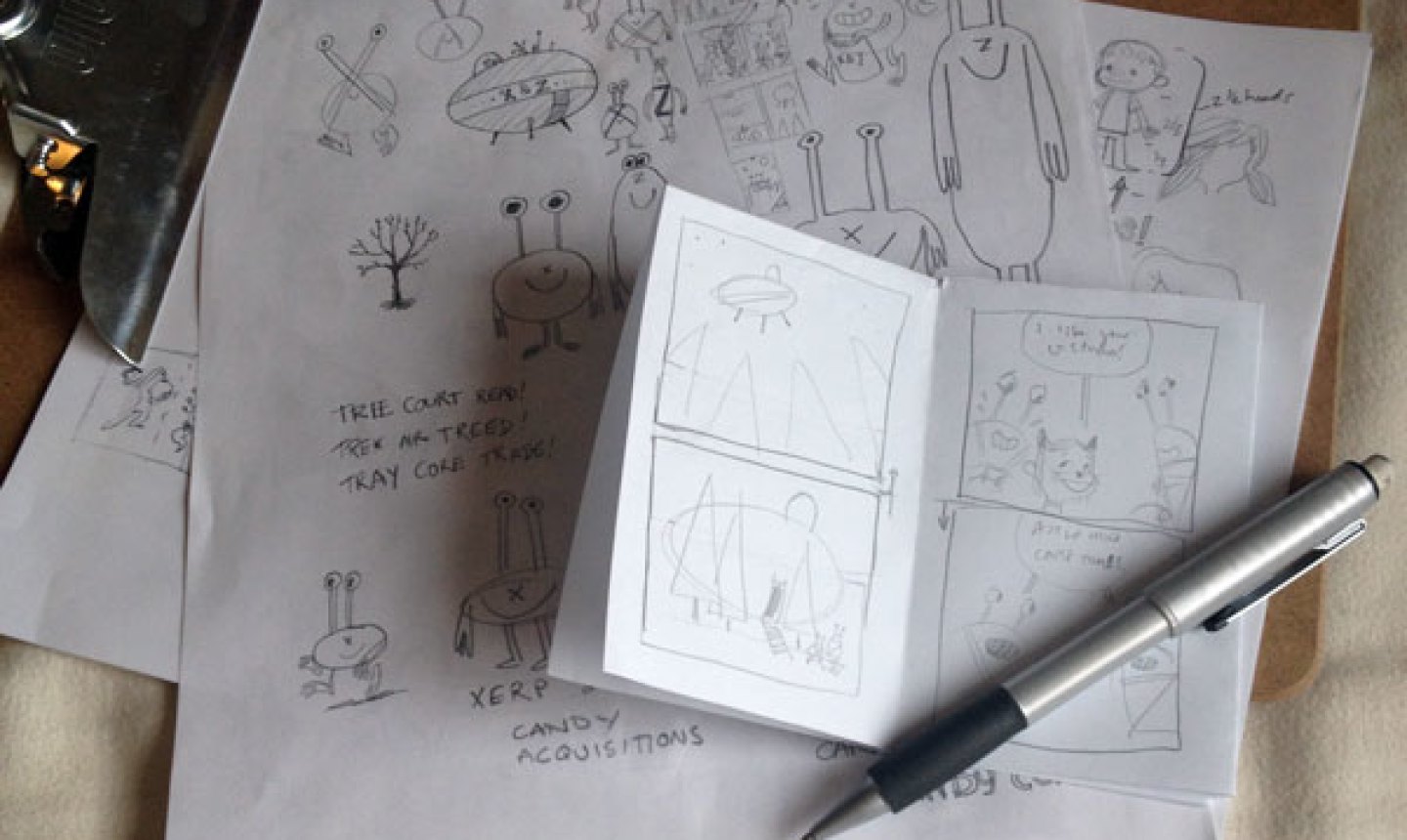The image captures a detailed scene of creative doodling and comic drafting. Centered on a brown clipboard with a metal clip, multiple white sheets of paper showcase a variety of black ink sketches. The top sheet, folded like a booklet, features four comic book-style panels illustrating a sequence involving spaceships, aliens, and interactions with a character. The text in these panels is too small to read clearly. Below this folded booklet, other sheets contain numerous whimsical alien drawings, with creatures sporting antennae with eyes, short arms, and splendid legs. The term "candy acquisitions" appears in the text scattered across these drawings. In the bottom right corner of the image, a silver pen with a black ergonomic grip lies diagonally across the papers, suggesting active use in the doodling process. The entire assembly evokes the playful and imaginative efforts of someone, perhaps a child, crafting their own comic scenes. The setting rests on a soft, dark cream surface, providing a cozy backdrop to this burst of creativity.